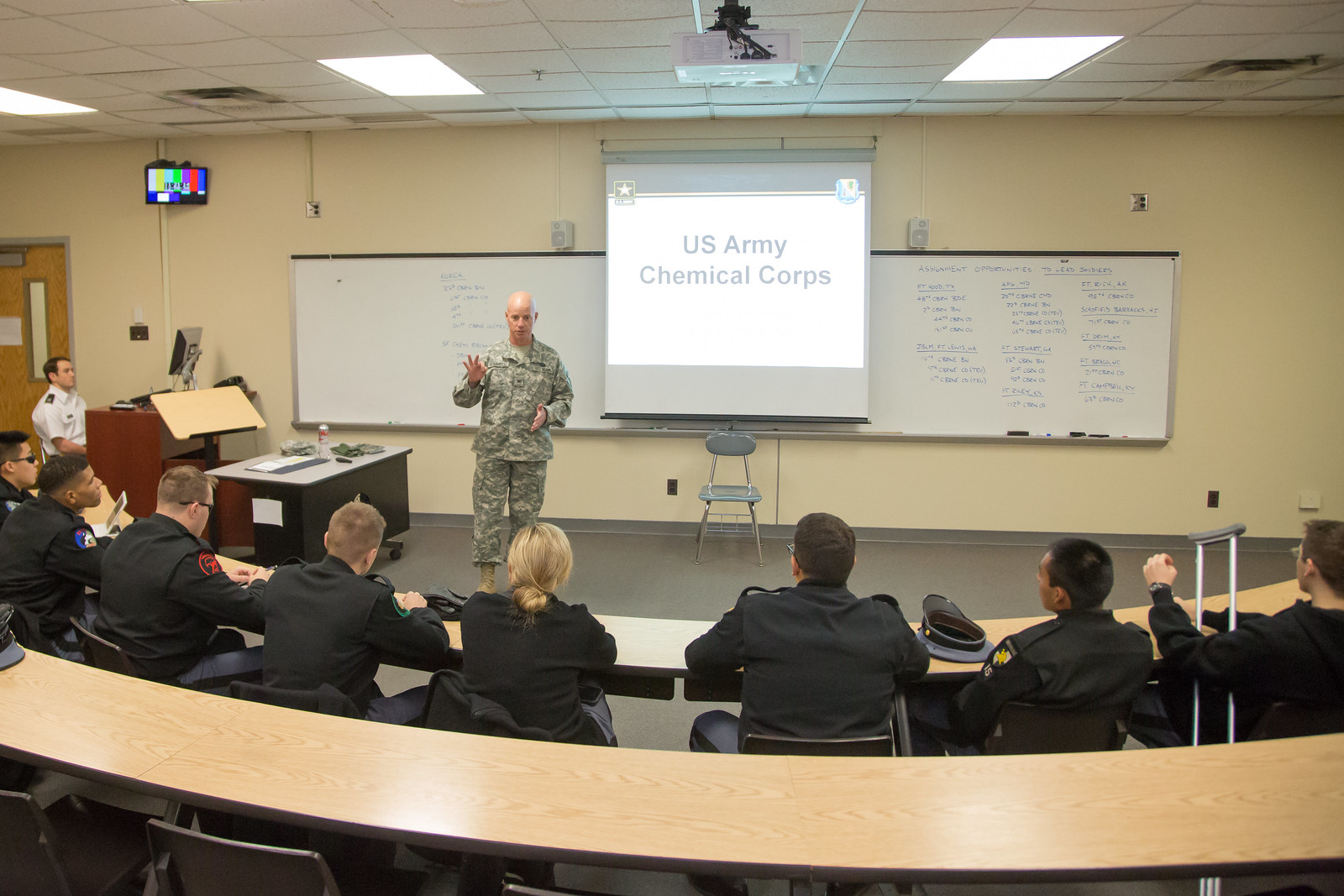The image captures an indoor setting resembling a classroom or training room, with a primary focus on a man in the center wearing army fatigues, including a camouflage jacket and pants, delivering a presentation. The man stands behind two long beige wooden desks, the one closest to the bottom of the image is empty, while the second desk in front of it is occupied by about eight young people. Most of these individuals, including a female, are dressed in black long-sleeve shirts, pants, and some wearing black jackets, appearing to be students or trainees. The floor they are sitting on is gray, and they are attentively watching the man in fatigues.

The background of the image features a beige wall adorned with a large rectangular dry erase board, some of which contains unreadable blue writing on the right-hand side. Hanging centrally above the dry erase board is a projection screen displaying the text "U.S. Army Chemical Corps." To the left of the man giving the presentation, there is another black and gray rectangular desk with various small items, including what looks like a keyboard. Additionally, on the left side in the background, a man in a white uniform sits at a brown desk, focused on a computer monitor. The image's color palette includes gray, light brown, black, red, blue, yellow, tan, green, white, purple, and pink, contributing to the detailed setting of what appears to be a military training event.